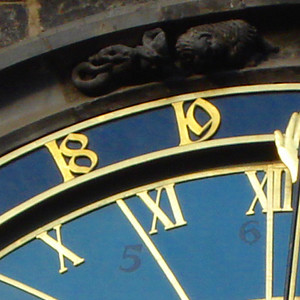This image is a very close-up photo of an ornate outdoor clock mounted on a dark brick or stone building, likely historic due to the stone embellishments and polished appearance. The clock face is predominantly blue with gold accents, including gold numerals and markers that are distributed in two layers: an outer layer showing 18 and 19, and an inner layer featuring Roman numerals X, XI, and XII, indicating 10, 11, and 12 o'clock. The visible portion of the clock, less than the top left quarter, highlights intricate detailing. Above the clock, there are carvings or sculptures of indeterminate animals, made indistinct by the lighting and resolution. The clock hand, positioned near the edge, is notable for its unique design, ending in what resembles an actual hand. The entire scene is set against a deep, royal blue backdrop, adding to the grandeur of the clock.